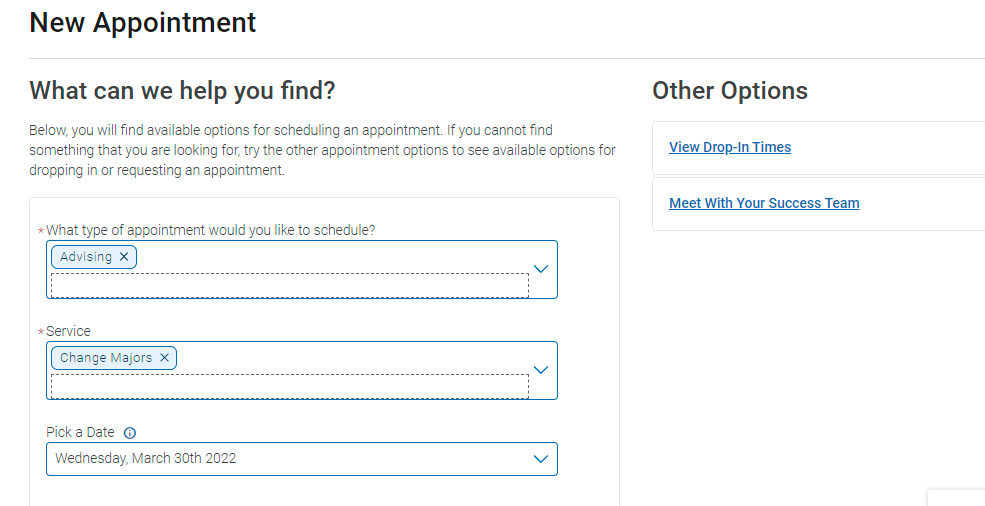The image appears to be a screenshot of a computer interface, primarily featuring black text on a white background. In the upper left corner, it bears the title "New Appointment," followed by the prompt, "What can we help you find?" Below this is a smaller instructional text that reads, "Below, you will find available options for scheduling an appointment. If you cannot find something that you are looking for, try the other appointment options to see available options for dropping in or requesting an appointment."

The interface is divided into three categories to fill in for scheduling:
1. Under the header "What type of appointment would you like to schedule?", a blue box labeled "Advising" is present next to a corresponding empty selection box.
2. The next section, titled "Service," features another blue box with the label "Change majors."
3. The final section, "Pick a date," indicates the date "Wednesday, March 30th, 2022."

On the right side of the image, prominent black letters spell out "Other Options." Below this heading, in blue text, are links that say "View drop-in times" and "Meet with your success team."

The overall context suggests that this interface is used for scheduling appointments within a college setting, likely for consultations with academic advisors or guidance counselors.